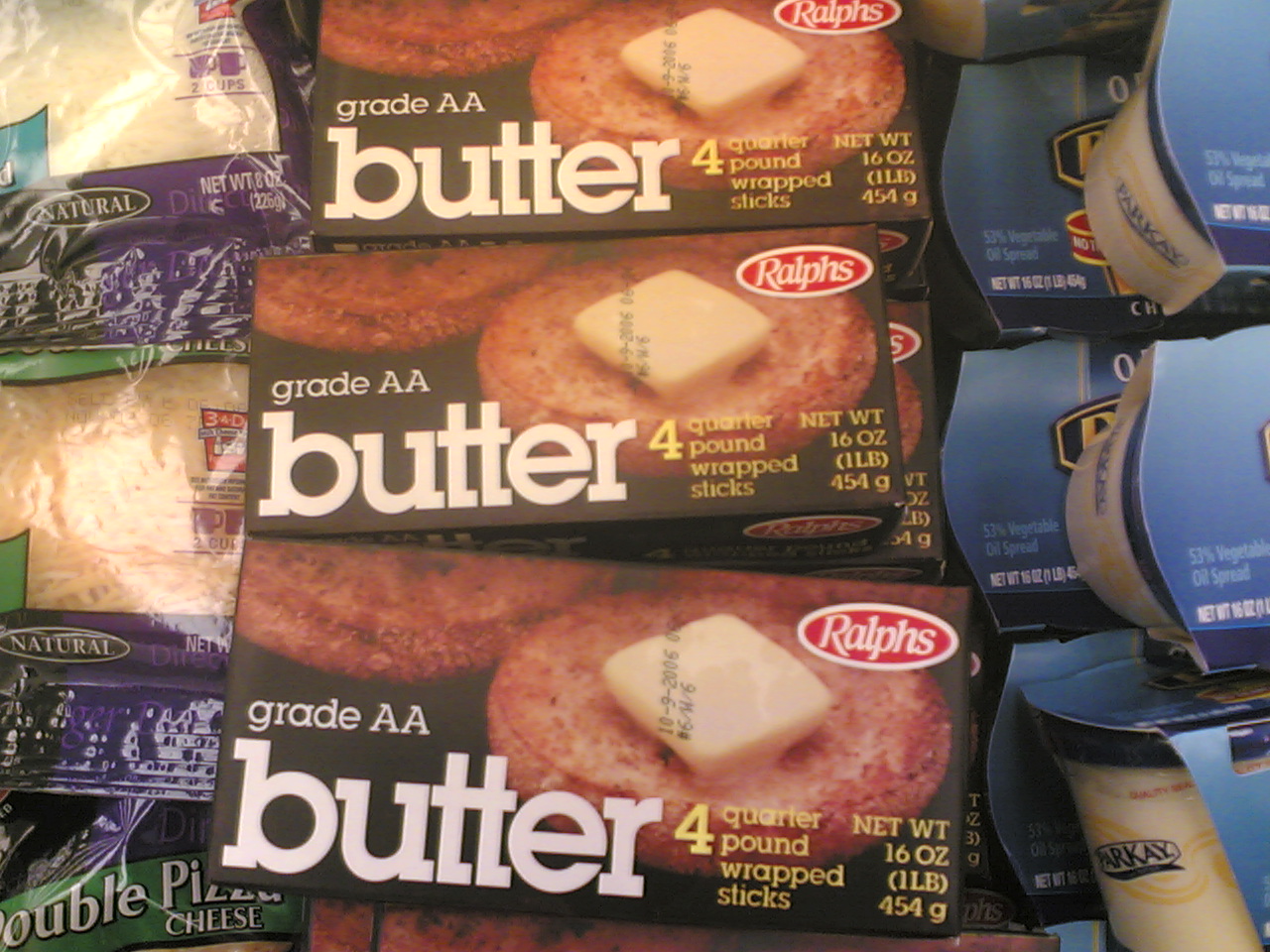In this detailed image of a grocery store section, three distinct items are prominently displayed. On the left, there is a bag predominantly colored in purple and green, featuring a transparent section in the center that reveals shredded cheese inside. The bag is labeled with the word "Natural" at the bottom. Adjacent to this is a product with a green label embossed with white text that reads "Double Pizza Cheese." To the right, there is a black box that sports an image of bread with butter spread on it. The box bears the brand name "Ralph's" in red and white, along with the description "Great Double A Butter," and contains four quarter-pound wrapped sticks of butter. Finally, on the far right, there is a blue box housing containers in red, white, blue, and yellow, all branded with the name "Parquet."